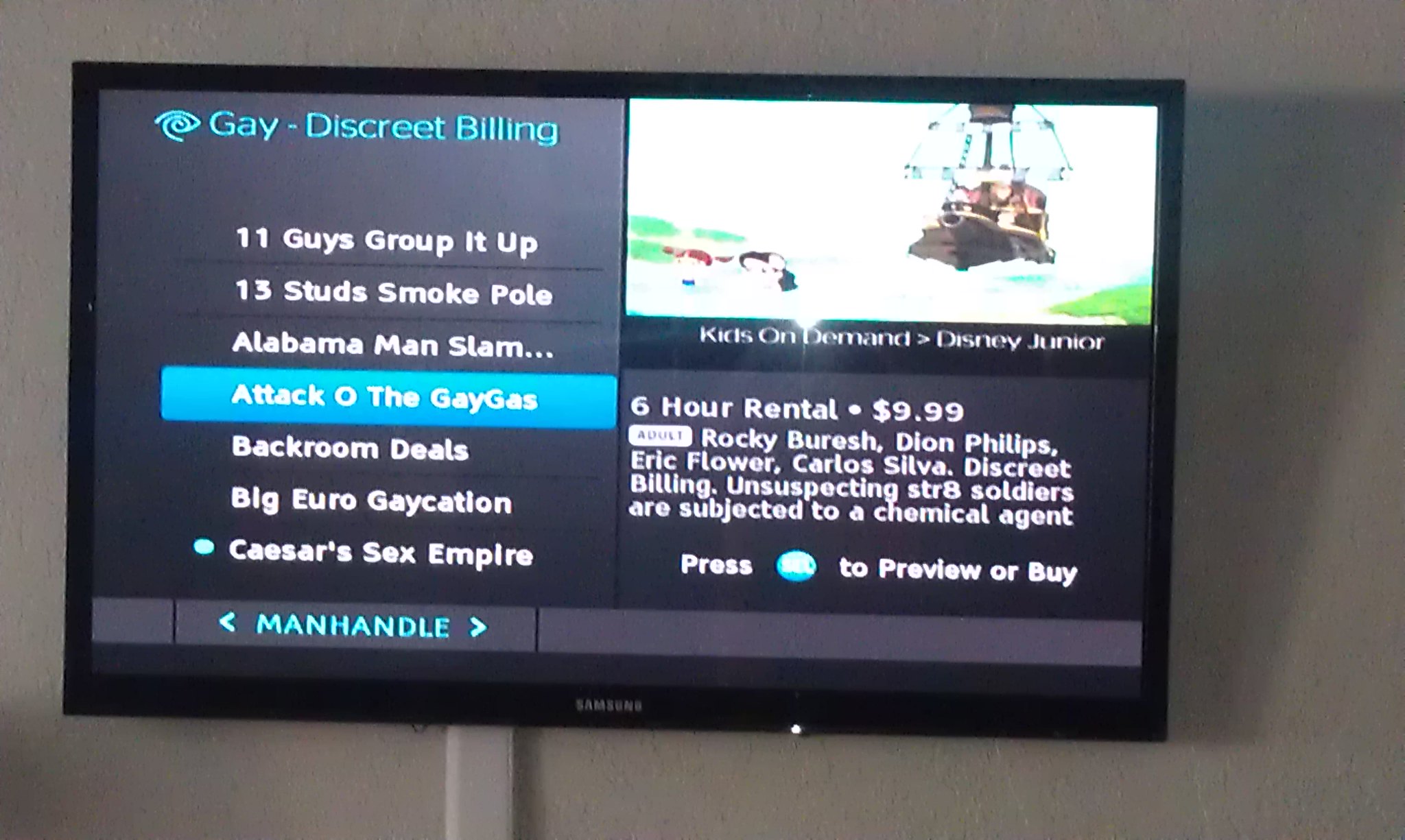The image showcases a Samsung TV with a black border mounted on a white, textured wall, likely in a hotel room. The screen is split into two distinct sections. The left half is dedicated to gay adult movie rentals, prominently featuring titles such as "11 Guys Group It Up," "13 Studs Smoke Pole," "Alabama Man Slam," "Attack of the Gay Gas," "Backroom Deals," "Big Euro Gaycation," "Caesar's Sex Empire," and "Manhandle." Each title is accompanied by the text "Gay - Discreet Billing," emphasizing anonymity. Also listed are the names Dion Phillips, Eric Flower, Carlos Silva, and other actors. In stark contrast, the right half of the screen displays content catered to children, including a Disney Junior show titled "Rocky Buresh," available for a six-hour rental at the cost of $9.99. The image highlights the bizarre juxtaposition of adult content alongside a Disney children's program, underlining the unusual and somewhat disconcerting nature of the offerings. At the bottom of the screen, users are prompted to "Press to Preview or Buy" either type of content.